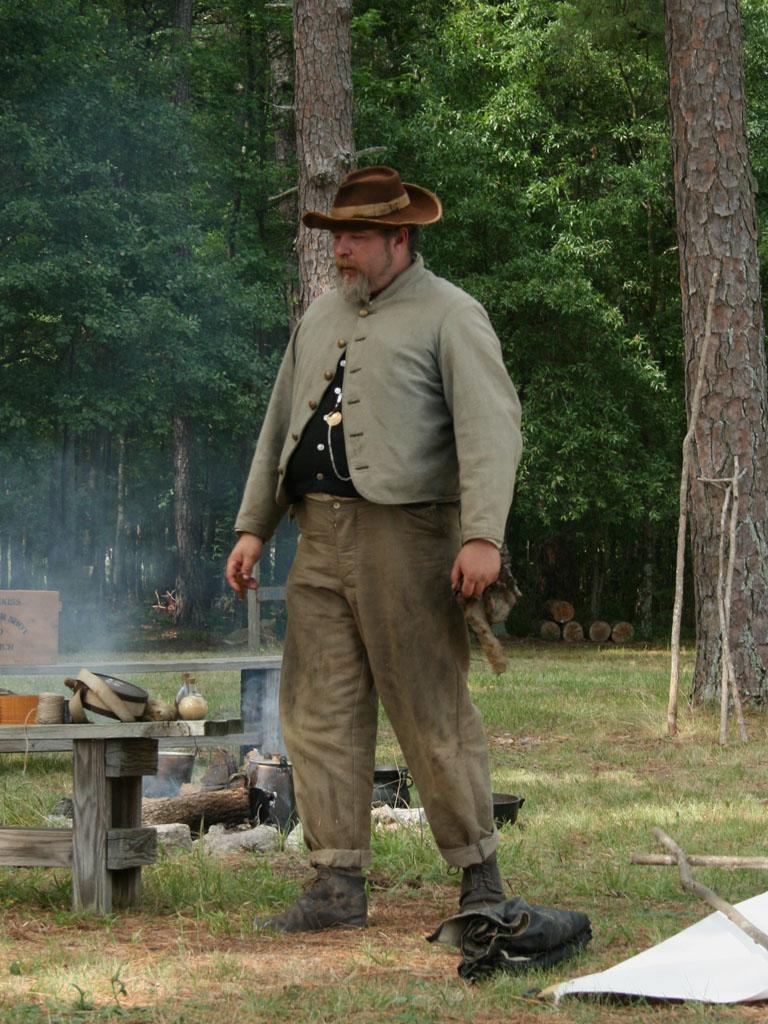In the image, a man is seen standing outdoors, facing towards the lower left side of the frame, allowing a view of both his front and left profile. He is dressed in rolled-up brown pants and sturdy brown boots, suggesting a rugged, outdoor activity. The man dons a gray shirt layered over a black button-down shirt underneath, with the gray shirt left open towards the bottom. His attire is completed with a brownish hat atop his head and a thick goatee that is notably longer around the chin area. The surroundings include an outdoor setting featuring a picnic table and a small fire pit bordered with stones, reinforcing the casual, rustic atmosphere of the scene.